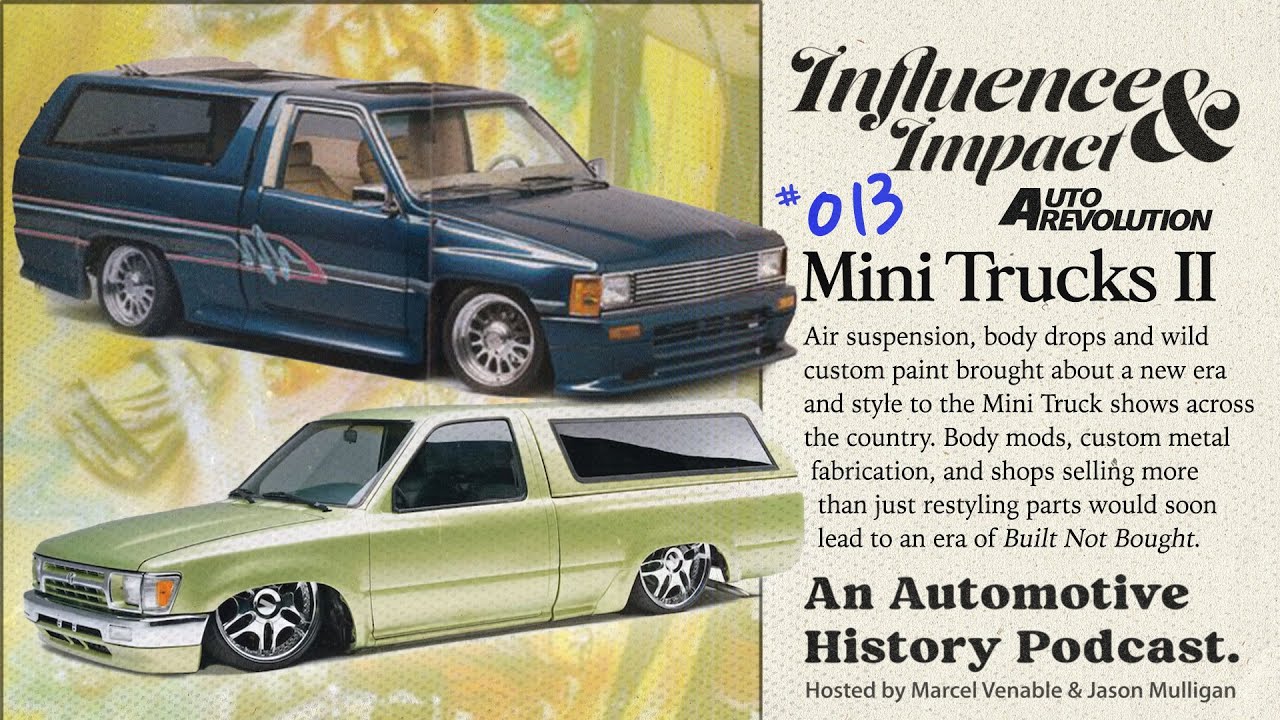This is a horizontally aligned rectangular graphic design image featuring two older style mini trucks on the left and informational text on the right. The mini trucks have a retro feel, with the one on top being a dark navy blue adorned with fuchsia and light blue stripes, while the one on the bottom is a bright green. Both trucks are low to the ground and have campers attached to their backs.

The background behind the vehicles incorporates shades of yellow and brown and vaguely suggests a person's face, adding a vintage touch to the overall aesthetic. On the right side, there is a series of texts explaining the significance of these vehicles. At the top, large bold letters state "Influence and Impact," followed by "Auto Revolution" in dark brown text. Below, handwritten in blue, is "#013." The primary paragraph beneath this heading reads, "Mini Trucks II: Air suspension, body drops, and wild custom paint brought about a new era in style to the mini truck shows across the country. Body mods, custom metal fabrication, and shops selling more than just restyling parts would soon lead to an era of built, not bought." 

The bottom of the text features large, bold brown letters that state, "An Automotive History Podcast," followed by "Hosted by Marcel Venable and Jason Mulligan."